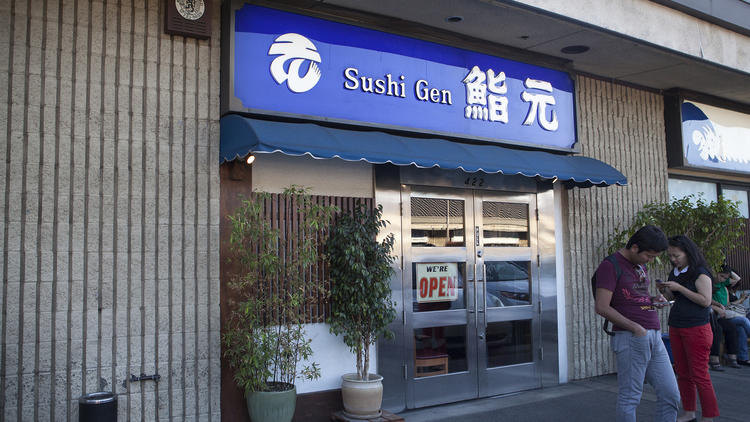The image depicts the inviting storefront of a sushi restaurant named Sushi Gen, distinguished by its gray stone walls and stainless steel double doors with multi-pane glass windows. Above the entrance, a vivid blue awning with a white border draws the eye, further complemented by a blue sign that reads "Sushi Gen" in English, flanked by Japanese characters. The facade features potted plants in tan ceramic pots on either side of the doorway, adding a touch of greenery. To the left of the door stands a black ashtray with a silver top. The scene captures three individuals: a man in a red shirt and gray pants and a woman in a black shirt and red pants, both focusing intently on their phones. In the background, partially obscured by foliage, a man in a green shirt sits on a bench, also engaged with his phone. A "We’re Open" sign is visible through the door’s glass panes, welcoming patrons inside. The edge of an adjacent storefront is faintly seen to the right, under the building’s slight overhang.